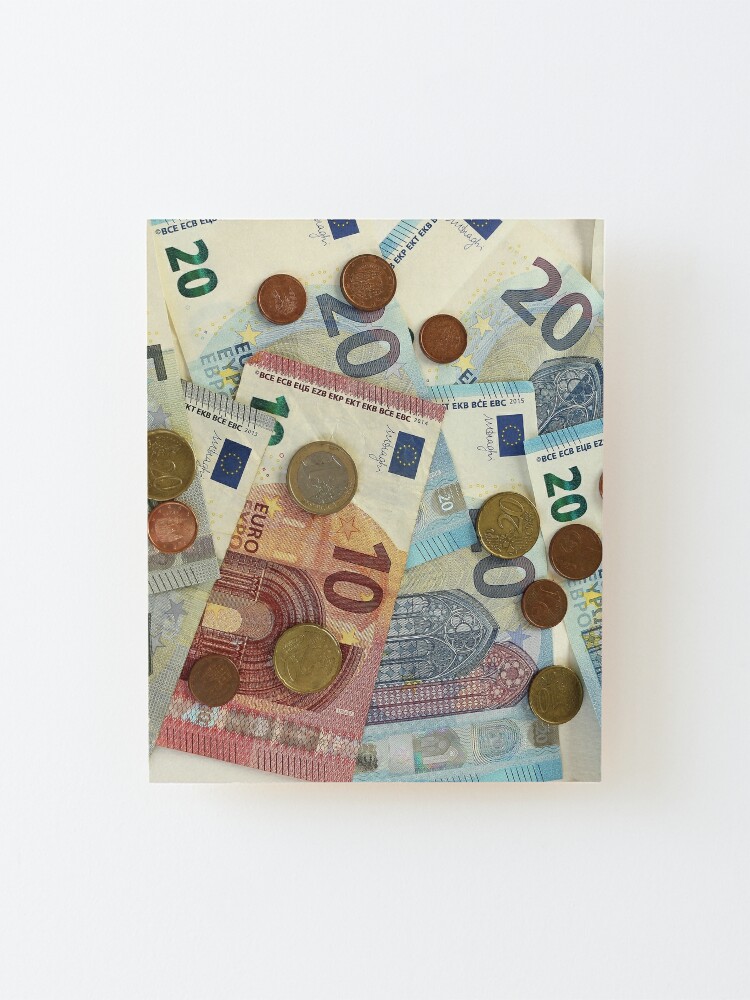From a top-down perspective on a white table, the image showcases a vibrant assortment of monetary units, highlighting both paper bills and coins. The paper bills are scattered in a seemingly haphazard manner, consisting predominantly of 20 and 10 denominations. The bills vary in color, featuring shades of green, blue, and red. Notably, one of the red 10 bills is identified as a euro, suggesting the presence of various European currencies, though some are unfamiliar to the viewer. 

The arrangement includes numerous coins of differing sizes and shapes, prominently gold, bronze, copper, and silver in color. Among these, a gold coin clearly displays the number 20, while others are less distinct. The coins rest atop the paper bills, adding a textural contrast. The 20 bills are primarily in lighter and darker blue hues, while the 10 bill appears light pink or maroon. 

The entire mix is encased in a square in the middle of a gray background, framing the colorful and somewhat chaotic presentation of currency. The composition includes one bill with a slightly upturned corner, adding a subtle note of imperfection to the orderly yet random layout.